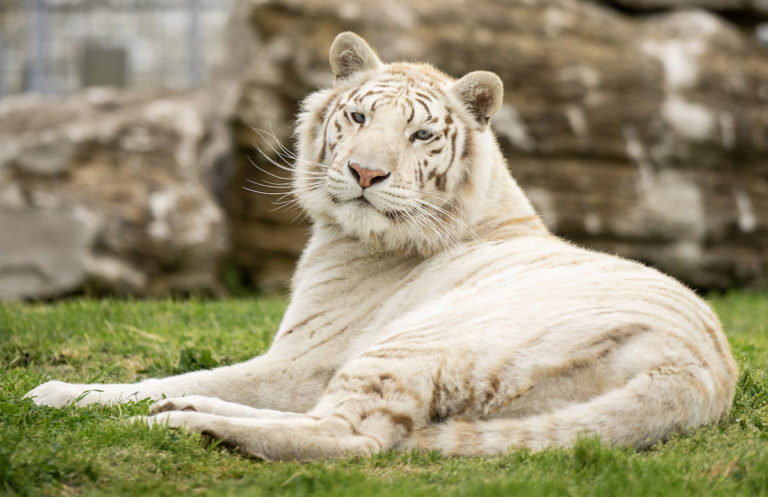The image captures a serene scene of a relaxed white tiger with light brown stripes, lying on a green, grassy field. The tiger, with its pink nose and prominent white whiskers, looks directly at the camera with half-closed eyes, suggesting a state of calm contentment. The background features a blurred stone wall or natural rock structure with blackish and brownish hues, and in the top left corner, there is a faint outline of a fence or gate, hinting at a controlled environment like a zoo. The entire scene is dominated by the majestic tiger, whose large, graceful presence and almost smiling expression embody tranquility.